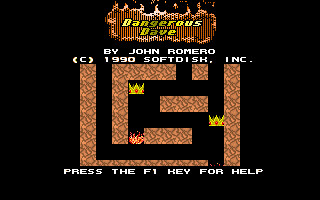An image of a retro video game screen on a black background. At the top, a pixelated oval with flames, labeled "Dangerous Dave" in yellow text, is prominently centered. Below this, white text credits "by John Romero," with a copyright notice stating "circa 1990 Softdisk Inc." The screen's lower portion showcases a brown, pixelated maze, giving a rustic, rocky appearance. In the maze, there are notable placements of crowns in the top left and center-right corners, along with a fire icon in the bottom left path. At the very bottom, instructions read, "Press the F1 key for help." This nostalgic game screenshot is characterized by its low resolution and retro style, typical of early 90s PC games.